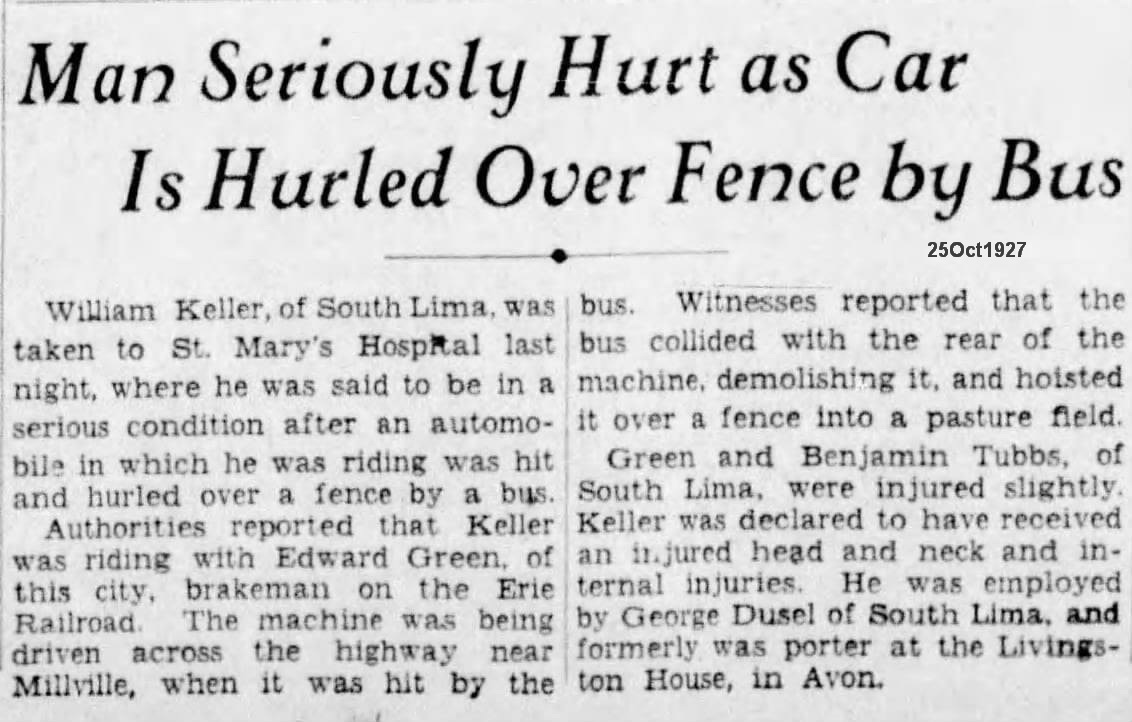The image depicts a light gray newspaper clipping with bold black text. The headline reads, "Man Seriously Hurt As Car Is Hurled Over Fence By Bus," dated 25 October 1927. The article details that William Keller of South Lima was taken to St. Mary's Hospital in serious condition after the car he was in was struck by a bus and thrown over a fence. Keller, riding with Edward Greene, a brakeman on the Erie Railroad, was crossing the highway near Millville when the bus rear-ended their vehicle, demolishing it and flinging it into a pasture field. Greene and another passenger, Benjamin Tubbs of South Lima, sustained minor injuries. Keller, who suffered head, neck, and internal injuries, was employed by George Dussel of South Lima and formerly worked as a porter at the Livingston House in Avon.